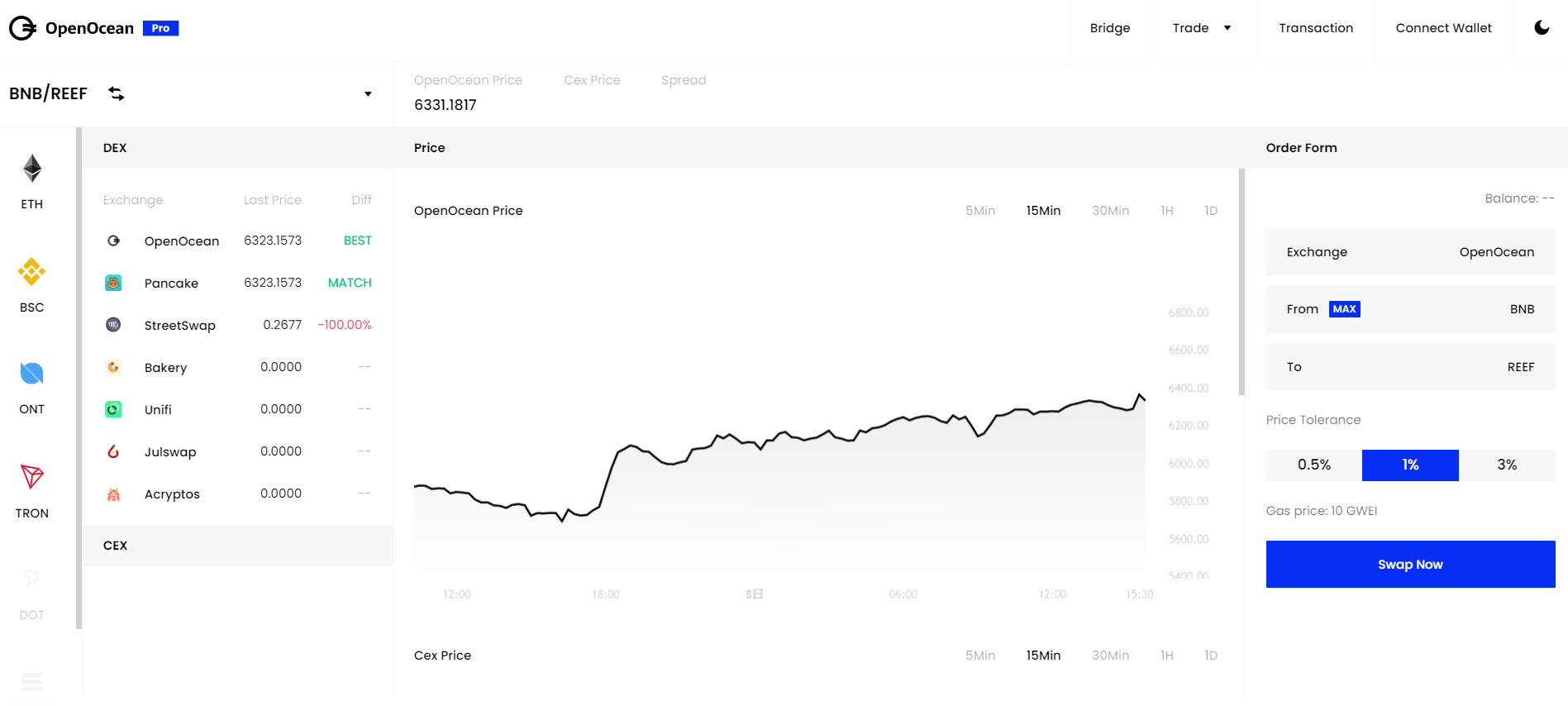Caption: 
A detailed screenshot of the OpenOcean website interface showcases a variety of options and tools available to users. On the right side, prominently featured are navigation tabs labeled "Bridge," "Trade," "Transaction," and "Connect Wallet," accompanied by a moon icon. To the left, there is a display for BNB/REF trading pairs, with a refresh symbol adjacent. This symbol is designed as an arrow pointing to the right overlain by an arrow pointing to the left.

The website supports multiple blockchain networks indicated by the labels: ETH (Ethereum), BSC (Binance Smart Chain), CNT, and TRON. Additionally, the terms "Debts" and "Price" are noted, hinting at the financial functionalities provided.

A line graph is featured, tracking the price movement of OpenOcean. Adjacent to the graph, there is an order form section accompanied by options for "Exchange" and "Balance." Under the "Balance" section, the platform lists "OpenOcean," with options to exchange "from" a maximum value, highlighted in white text on a blue rectangle, "Max."

At the bottom of the interface, a prominent blue rectangle with white text invites users to "Swap Now," encouraging immediate engagement in trading activities.